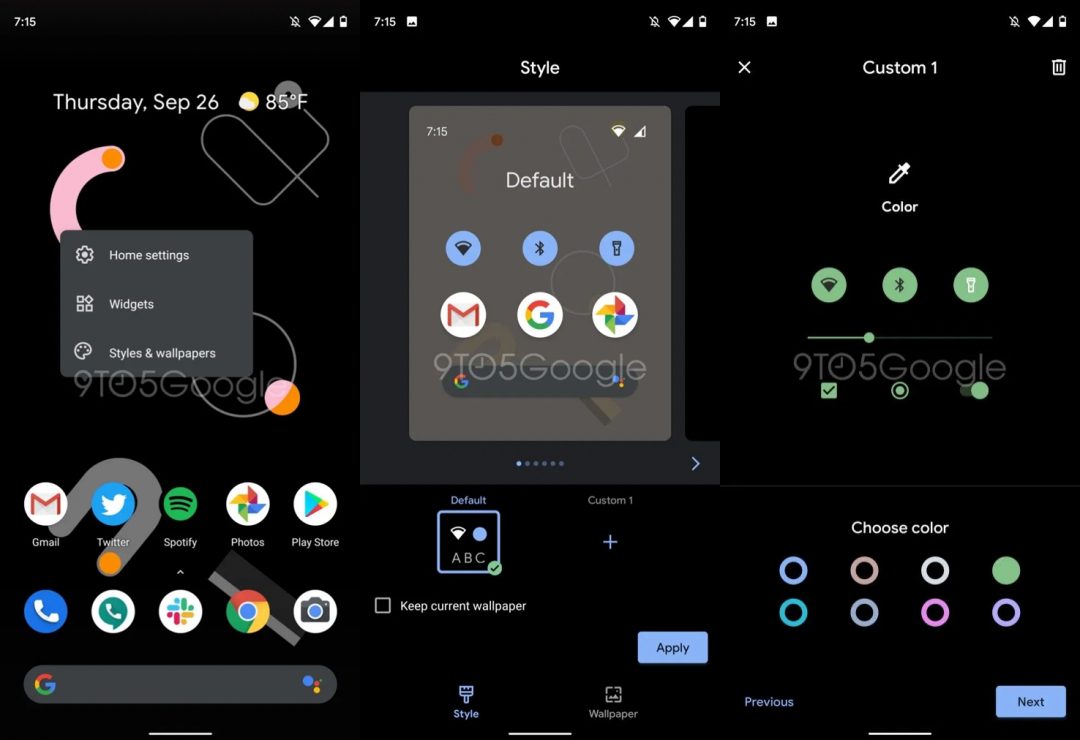The image is a collage of three phone screen captures, each with a black background, set side-by-side. All three screens display different home screens from mobile devices but share several common elements: 

- The top right corner of each screen shows a battery symbol indicating a charge level between half and three-quarters full, along with full cellular service bars.
- The Wi-Fi signals differ slightly; the rightmost screen shows a full Wi-Fi connection, while the center and left screens display one bar short of full connection. All screens have notifications silenced, as indicated by respective icons.
- In the upper left corner, the date "7-15" is consistently displayed across all three screens.
- Both the center and right screens feature a small picture icon at the top.

A distinctive watermark labeled "9T, a clock symbol, 5Google" is superimposed on each of the images.

- **Left Screen**: This screen shows the home menu with options for 'Home,' 'Widgets,' and 'Styles' visible above a grid of various app icons.
- **Center Screen**: The focus here is on a menu for changing the wallpaper. The current setting is 'Default,' and a prominent 'Apply' button is present in the corner.
- **Right Screen**: This screen showcases an interface for customizing icon colors, allowing users to select their preferred hues for the icons on their home screen.

The overall collage provides a detailed visual guide to customizing various elements of the device interface.